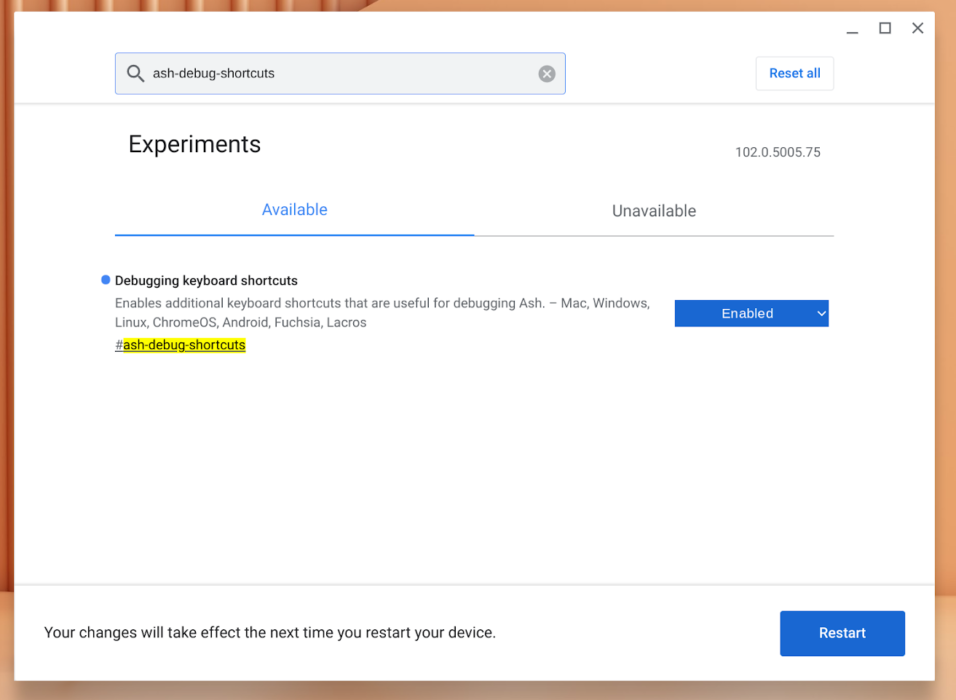The image shows a search bar at the top containing the text "ash-debug/shortcuts," with a magnifying glass icon on the left and a close button (X) on the right. Above the search bar, there are three icons: minimize (a dash), maximize (a box), and close (an X). Within a highlighted blue rectangle in the search results, the word "Reset all" is prominently displayed.

Below this, the screen is divided into three tabs: "Experiments," "Available," and "Unavailable," with the "Available" tab highlighted in blue. The section features a specific option titled "Debugging keyboard shortcuts," which enables additional keyboard shortcuts for debugging ASH. It mentions compatibility across multiple platforms: Mac, Windows, Linux, Chrome OS, Android, Fuchsia, and LaCrosse.

To the right of this description, there is an "Enabled" button in a blue rectangle with white text. At the very bottom of the interface, there's a notification in bold text stating, "Your changes will take effect the next time you restart your device." Right below this message is another blue rectangle button, this time labeled with the word "Restart" in white letters.